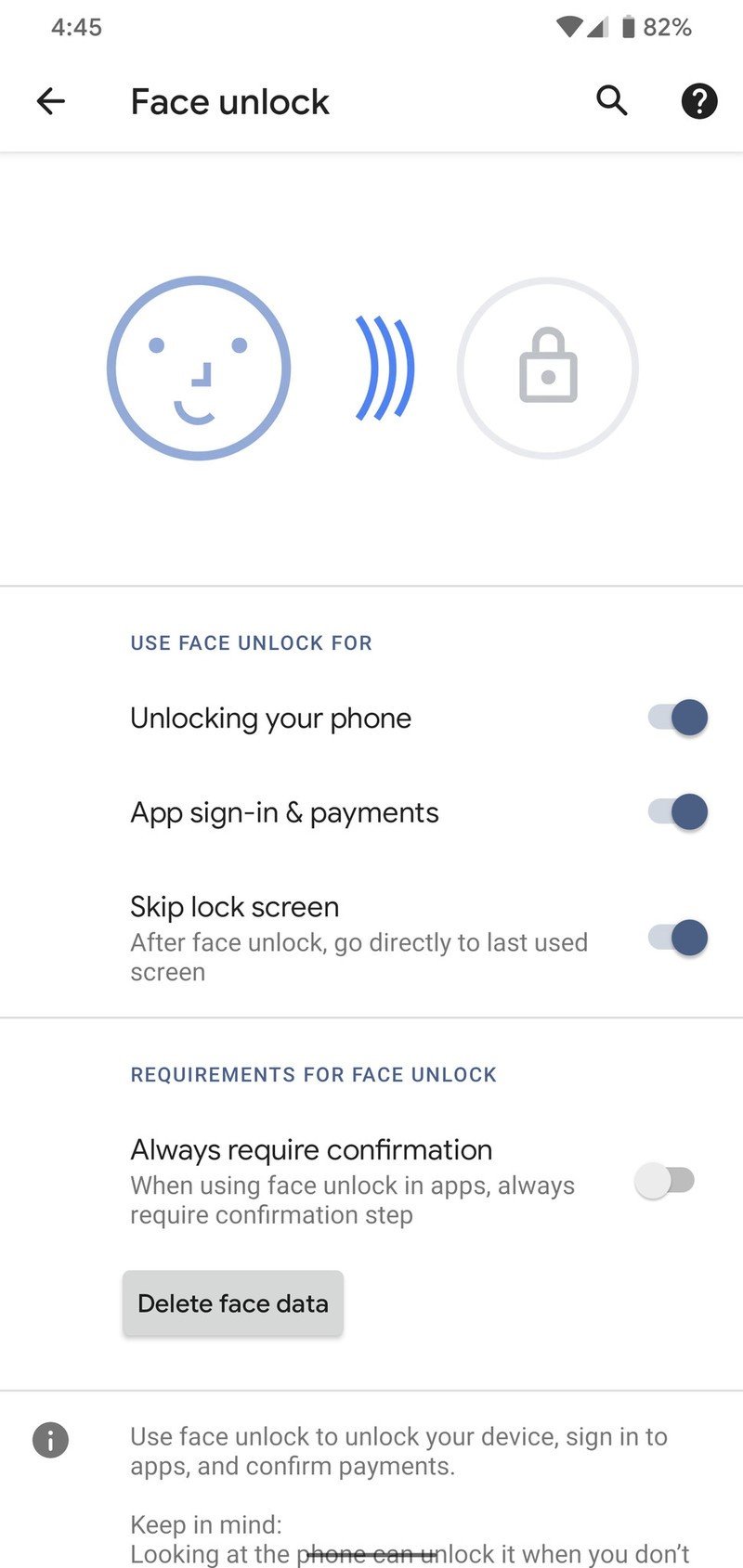Portrait-oriented color screenshot of a mobile phone settings page focused on face unlock feature. The device displays a time of 4:45 PM and shows 82% remaining battery life, with nearly full signal bars indicating strong internet reception. The highlighted section features a face unlock icon comprising a smiling face, a signal symbol, and a lock icon, indicating the feature is currently active but the phone is locked.

Key options with toggle switches beneath are visible, including:
1. **Use face unlock for unlocking your phone** - The switch is enabled.
2. **App sign-in and payments** - This option is turned on.
3. **Skip lock screen** - This feature is activated.

Below these primary options, there are additional settings under a section detailing face unlock requirements:
- **Always require confirmation** - Indicates a confirmation step is necessary when using face unlock within apps; this feature is currently disabled.
- **Delete face data** - A greyed-out button is available for deleting stored face recognition data.

The background of the settings page is plain white with standard black lettering, providing a clear and straightforward user interface.